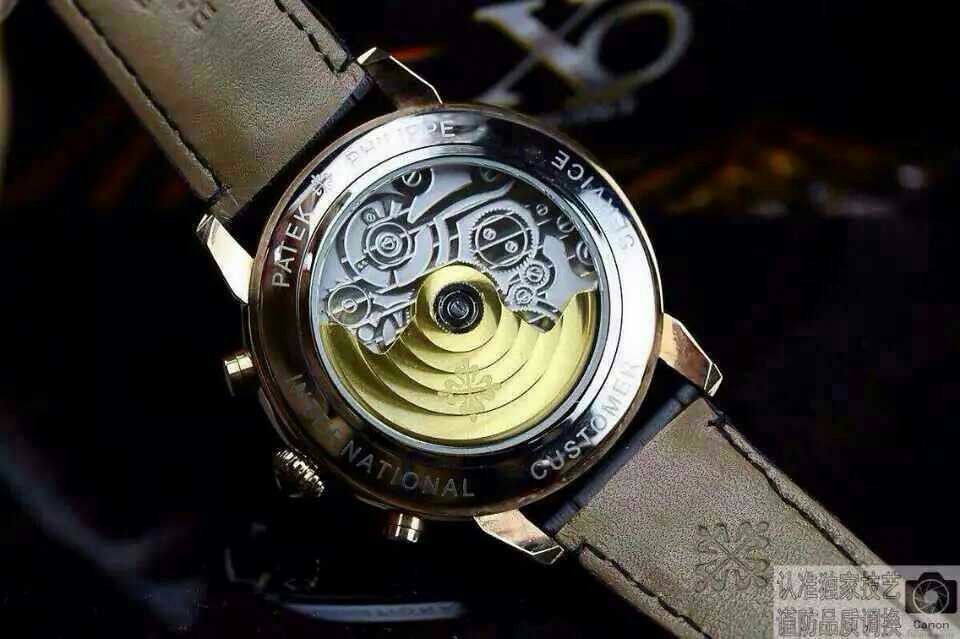A close-up image of a luxurious Patek Philippe watch, showcasing its exquisite craftsmanship. The watch features a pale gold bezel adorned with white engravings that detail various functions. The dial is intricately designed with terraced gold elements, adding a touch of ornate elegance. The strap is made of finely-grained leather in a pale grey color, accentuated with brown stitching, enhancing its sophisticated appearance. Several adjustment knobs are visible on the left-hand side of the watch, enabling precise settings. The watch is expertly illuminated, standing out vividly against a dark background, highlighting its opulent details and superior quality.